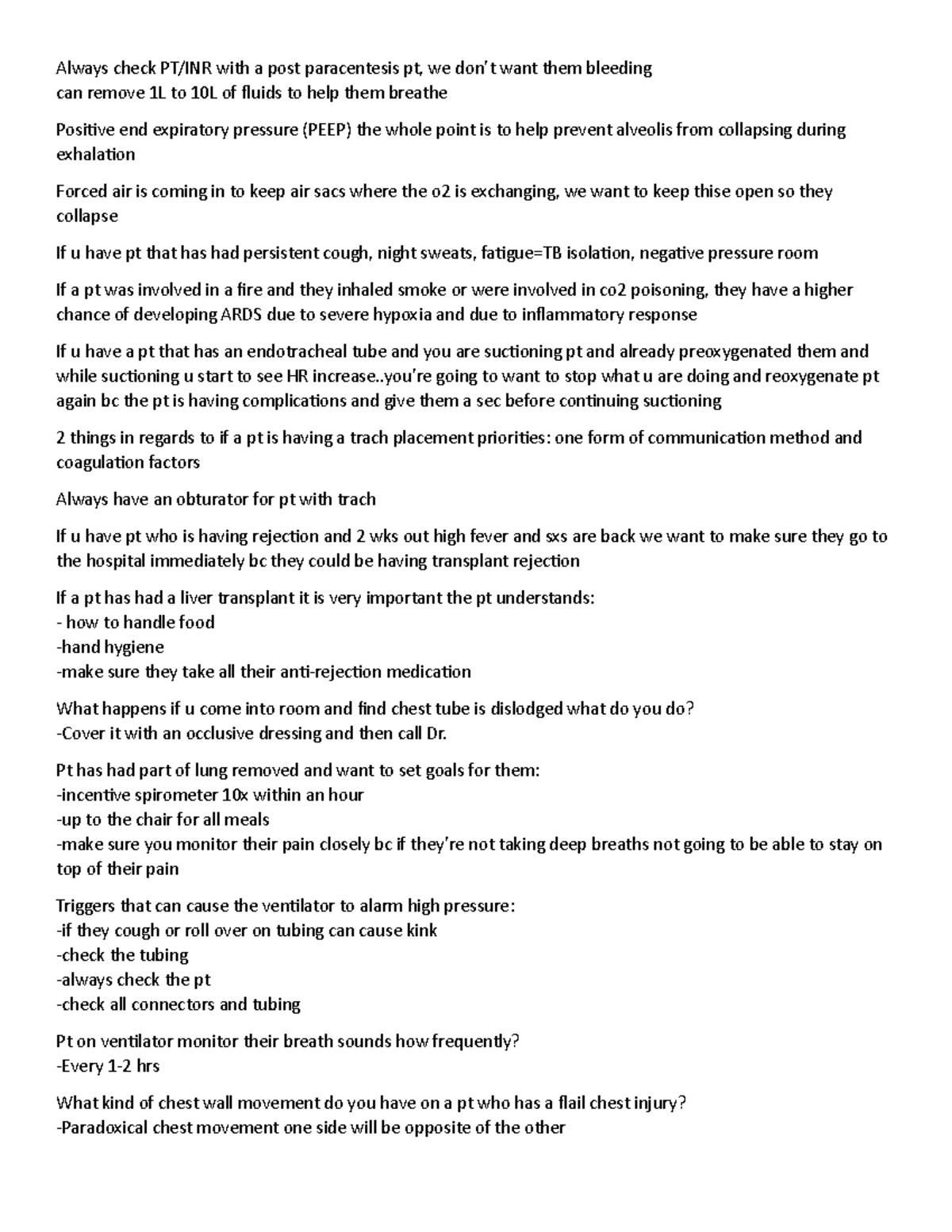This detailed caption elaborates on a range of healthcare guidelines and steps to follow concerning patient care, especially in critical situations. Below is a meticulously cleaned and descriptive caption:

---

"This image displays an extensive set of guidelines on patient care related to respiratory conditions and post-operative management. The text begins with the crucial reminder to always check PT/INR (prothrombin time/international normalized ratio) after procedures like post-paracentesis to ensure the patient does not experience bleeding. The guidelines suggest that removing 1L to 10L of fluids can aid in the patient's breathing.

There are instructions regarding the use of PEEP (positive and end expiratory pressure), which is pivotal in keeping alveoli open during exhalation to prevent lung collapse. Information is provided on managing patients with persistent cough, night sweats, and fatigue, indicating the need for TB isolation in a negative pressure room.

Special attention is given to patients who have been involved in fire incidents or CO2 poisoning, as they have a higher risk of developing Acute Respiratory Distress Syndrome (ARDS) due to hypoxia and the inflammatory response. For patients with an endotracheal tube, if heart rate increases during suctioning (even after pre-oxygenation), it’s crucial to stop and re-oxygenate before proceeding to prevent complications.

Additional guidelines focus on trach placement priorities, ensuring proper communication methods, and monitoring coagulation factors. If a PT shows signs of rejection such as high fever and recurring symptoms within two weeks post-transplant, immediate hospital admission is necessary due to potential transplant rejection.

For liver transplant patients, it is essential they understand handling food, maintaining hygiene, and adhering to their anti-rejection meds. Immediate action is recommended if a chest tube becomes dislodged, including covering with an occlusive dressing and notifying a physician.

Post-lung surgery goals include using an incentive spirometer 10 times per hour, sitting up for all meals, and closely monitoring pain management to facilitate deep breathing. Lastly, the text addresses ventilation alarms, emphasizing the importance of checking for high pressure causes like coughing or kinks in tubing, and ensuring regular monitoring of breath sounds every 1 to 2 hours. Recognizing paradoxical chest movement is critical in patients with a flail chest injury, where one side of the chest moves opposite to the other."

---